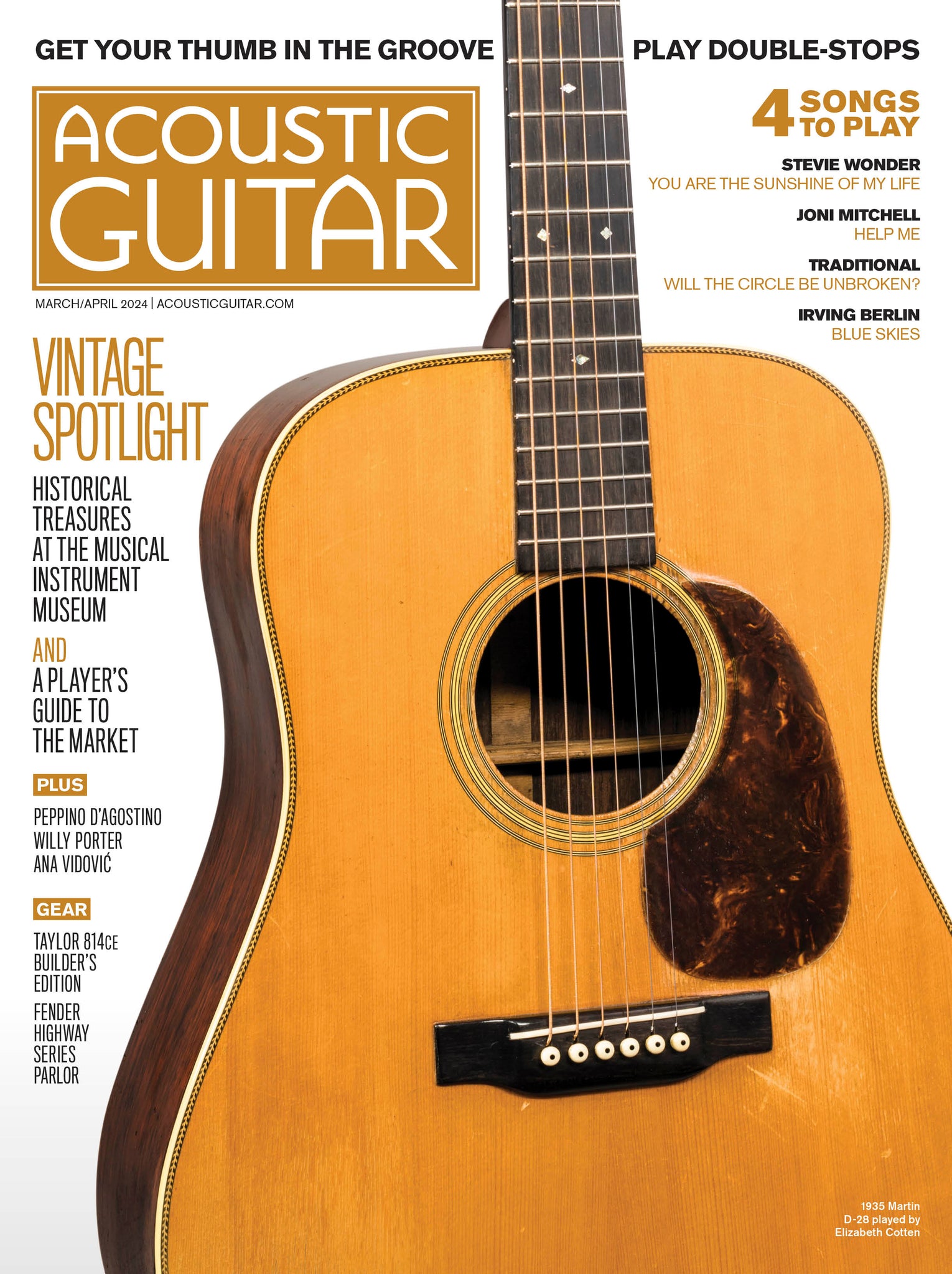This is a detailed color image of the cover of a magazine titled "Acoustic Guitar." At the top in black font, it says "Get Your Thumb in the Groove," while off to the right side, "Play Double Stop" is printed. Dominating the center is a large image of a guitar with a light wood face, dark wood sides, and a dark brown and light brown patterned protective plate. It features a dark brown neck with gold diamonds and six strings, each with white tuning knobs on the black headstock.

In the upper left corner, within a small light brown rectangle, "Acoustic Guitar" is written in white font. Below this, in smaller black and brown text, are the additional contents: "Vintage Spotlight: Historical Treasures at the Musical Instrument Museum," "A Player's Guide to the Market," and articles featuring "Pepino D'Agostino, Willie Porter, and Anna Vidovic." Gear reviews for "Taylor 814CE Builders Edition" and "Fender Highway Series Parlour" are also mentioned.

In the upper right corner, the magazine advertises "Four Songs to Play," including "Stevie Wonder's You Are The Sunshine Of My Life," "Joni Mitchell's Help Me," "Traditional Will The Circle Be Unbroken," and "Irving Berlin's Blue Skies."